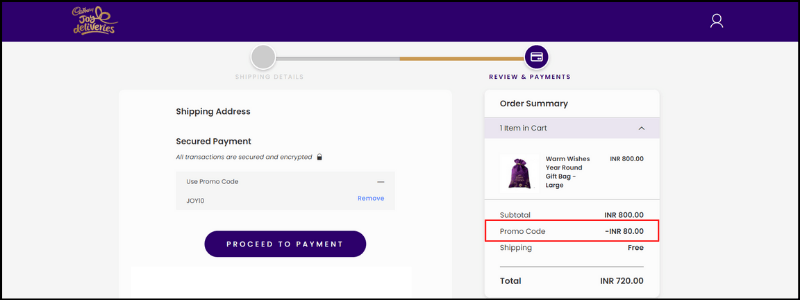The image is a detailed screenshot of a checkout page for Goldbug Deliveries. At the top, there's a prominent blue bar displaying the company name. Below it, a progress bar indicates the user's progress, showing "Shipping Details" grayed out, and "Shipping Review and Payments" highlighted in gold. 

Further down, there are sections labeled "Shipping Address," "Secured Payment," and text reassuring users that "All Transactions are Secured and Encrypted," accompanied by a lock icon. There’s also an option to "Use Promo Code," with "JOYQ" currently applied.

In the "Order Summary" section, it lists one item in the cart: "Warm Wishes Year-Round Gift Bag, Large." The item is priced at INR 800. The subtotal is also INR 800, but with the promo code "INR80," the total is reduced, and shipping is free, bringing the final amount to INR 720.